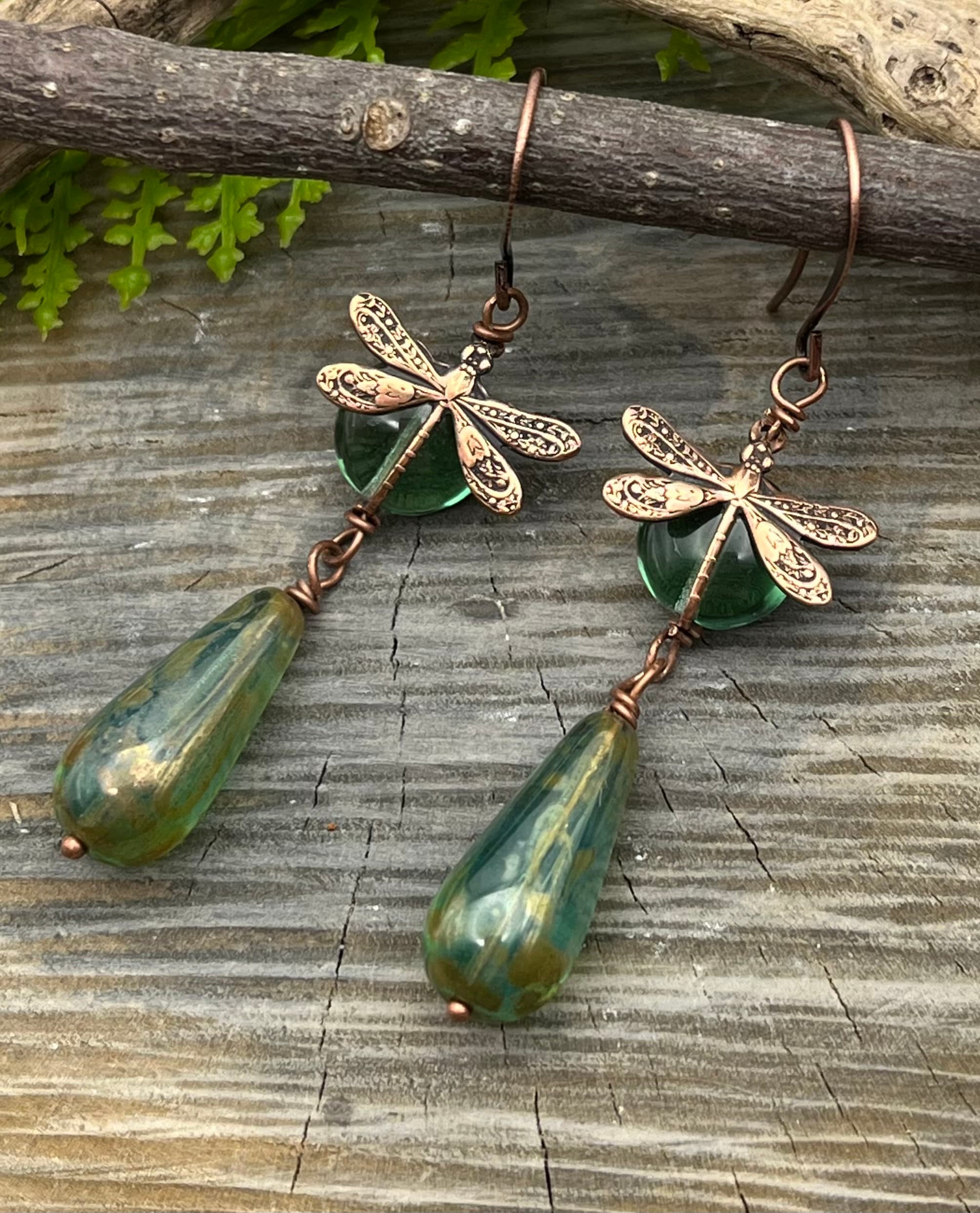The full-color vertical photograph, taken outdoors, features a detailed and artistic view of a rustic wooden table or countertop, its grain and numerous cracks adding texture to the setting. Strewn across the top are a few slender branches adorned with green leaves in the upper left corner. Draped over one of these branches is a pair of earrings. The earrings, possibly mistaken for wind chimes due to their intricate design, display a captivating combination of elements. Each features a bronze hook suspending a clear, green glass ball, adorned with a delicate golden dragonfly. Below this, a large, teardrop-shaped green stone, reminiscent of a bulb with a metallic base, hangs elegantly, completing the ornament. The overall composition brings together nature and craftsmanship, with the wooden backdrop and branches enhancing the earrings' aesthetic appeal.